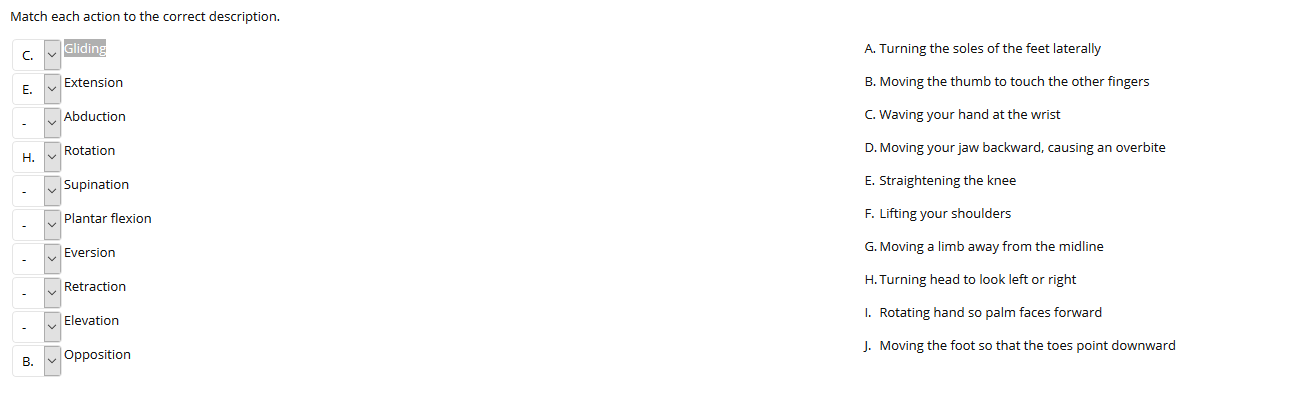The image features a predominantly white canvas that is significantly wider than it is tall, with its width roughly estimated to be three to four times its height. The layout consists of two distinct columns; the left column is aligned to the left side of the image while the right column is pushed towards the right side, though not strictly right-aligned.

In the left column, there is a black text prompt that reads, "Match each action to the correct description," and below it are several drop-down boxes, each corresponding to different letters. The text is completely devoid of color, ensuring a monochrome appearance.

The listed terms in the drop-down boxes on the left column include: 
- Gliding
- Extension
- Abduction
- Dislocation
- Supination
- Plantar Flexion
- Eversion
- Retraction
- Elevation
- Opposition.

Of these, only the entries corresponding to the letters C, E, H, and B have been filled. The entries are filled as follows:
- C
- E
- H (notably skipping the third entry)
- B (appearing in the last box).

The right column consists of descriptions corresponding to these actions, listed from A to H:
- A: Turning the soles of the feet laterally
- B: Moving the thumb to touch the other fingers
- C: Waving your hand at the wrist
- D: Moving your jaw backwards, causing an overbite
- E: Straightening the knee
- F: Lifting your shoulders
- G: Moving a limb away from the midline
- H: Turning your head to look left or right.

Overall, the image appears to be part of an anatomy exercise, focusing on matching specific movements or actions to their anatomical descriptions.